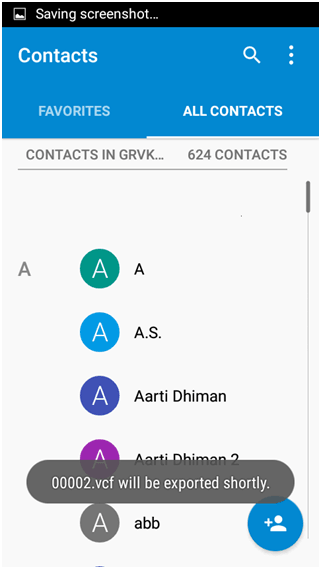The screenshot displays the contacts page of a phone. At the top, a slim black bar with white text and a small icon of a white square outline with a bit of a landscape indicates that the screenshot is being saved. Below this, a large blue rectangle prominently displays the word "Contacts." Towards the right-hand side, a magnifying glass icon for search and a three-dot icon to open a menu are visible.

The screen features two tabs titled "Favorites" and "All contacts." In light gray text, it indicates "Contacts in G, R, V, K," with three dots following this notation, and mentions there are 624 contacts. A gray line beneath provides a clean separation before the list of contacts begins.

The visible part of the contact list starts with those whose names begin with the letter A. On the left-hand side, an A in gray marks this section. Five contacts are visible, each represented by colorful circles with the letter A in white text inside them:

1. An aqua circle for a contact simply named 'A'.
2. A light blue circle for 'A S'.
3. An alphabetic contact, 'RD Demon', with a darker blue circle.
4. A magenta circle for 'RD Demon 2'.
5. A gray circle for 'ABB'.

In the lower right-hand corner, an aqua button with a plus sign and a person icon serves the function of adding a new contact. Additionally, a gray status bubble overlay is positioned over 'RD Demon 2' and between this contact and 'ABB'. It extends across most of the lower portion of the screen and states in white text that "00002.VCF will be exported shortly."